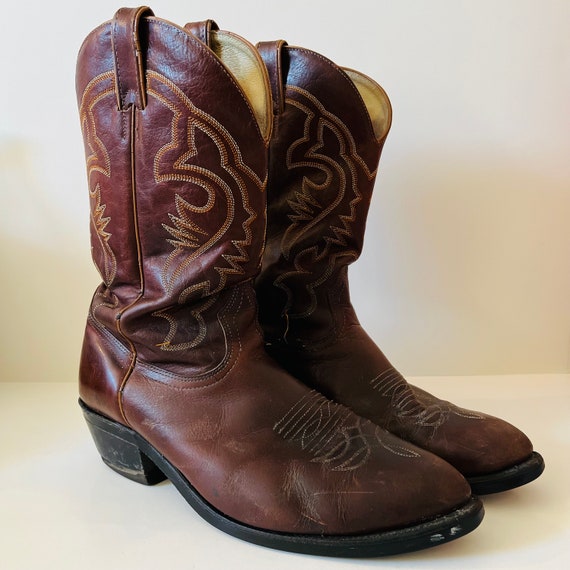This is a detailed product photo of a pair of very worn cowboy boots made of reddish-brown leather with a hint of burgundy. The boots, designed for durability and riding, have the traditional pointed toes and are elevated at the heels to fit into stirrups. Ornate stitching and etching adorn the uppers and tops of the toes, adding an intricate touch to their rugged appearance. The boots feature hand pulls at the tops and a noticeable side seam on the left boot. Despite their wear, evidenced by scuff marks on the toes and center and scratches on the leather, their craftsmanship shines through. The black soles and heels contrast with the lighter, beige interior. The boots rest on a smooth white surface, set against a very pale, almost gray background, providing a simple and clean backdrop to highlight their design.